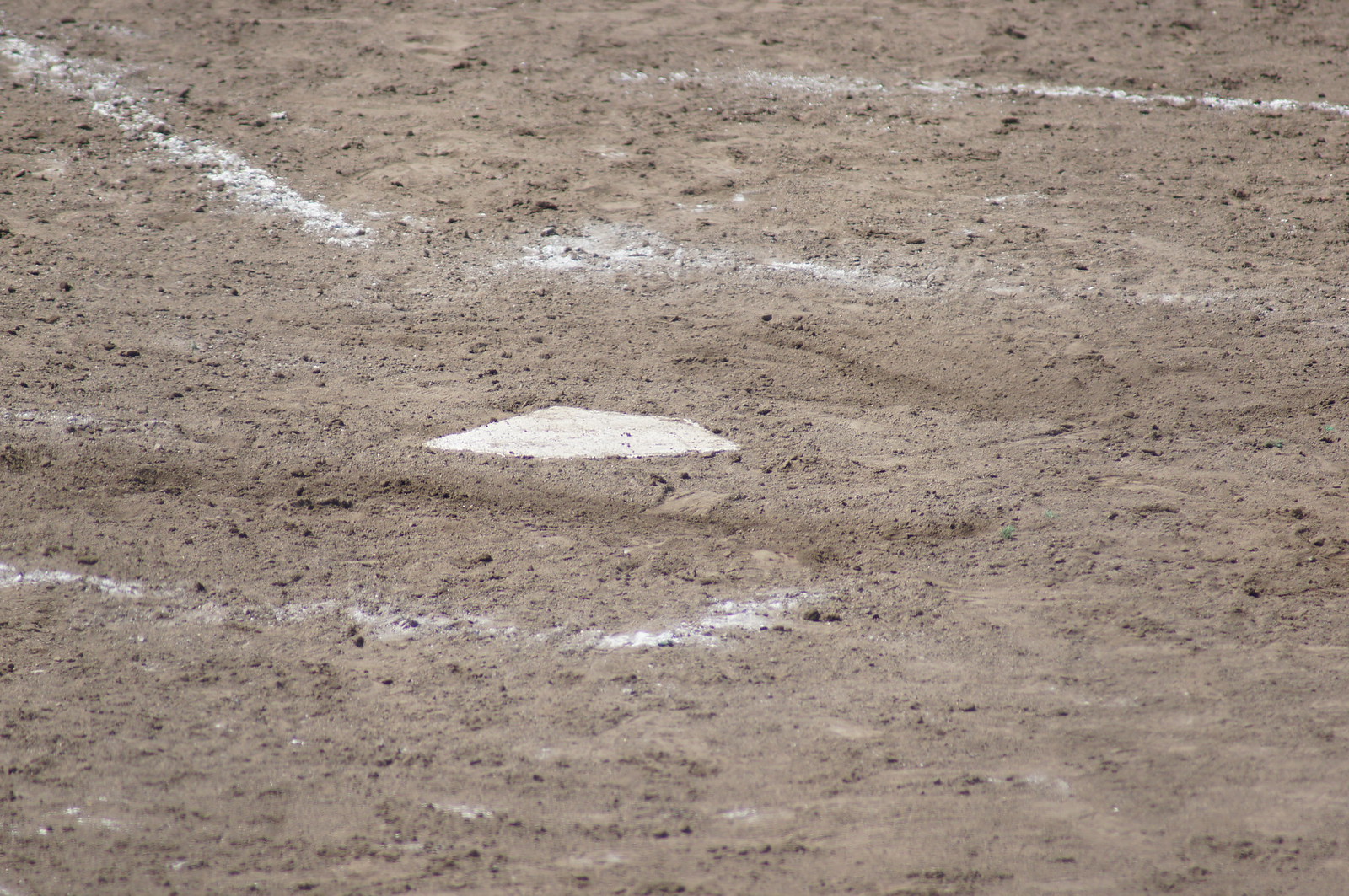This photograph captures a sunlit home plate on a baseball diamond. The home plate, predominantly white but speckled with dirt, is shaped with a squared back and a pointed front, lying just left of the center of the frame. The immediate surrounding ground consists of well-trodden, tan dirt, interspersed with rough, gravel-like pieces, displaying signs of heavy use with small hills and valleys indicative of both wear and possible rainfall. White chalk lines, drawn crisply, outline the base paths and create a distinct box around home plate. The vibrant image, taken from a distance, showcases these details clearly, emphasizing the purposeful markings and the textured, gritty terrain.